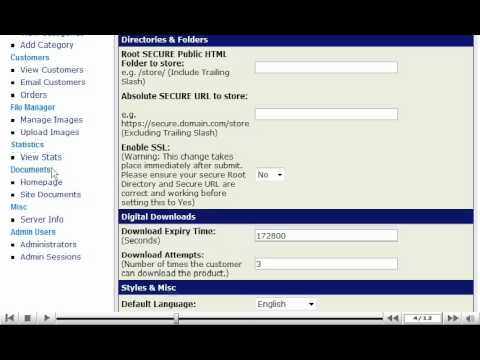The image portrays an administrative interface of a website's backend, which provides various tools and settings for managing the site. The layout consists of two primary sections, each framed by identical long, rectangular, black bars at the top and bottom. 

On the left side of the interface, there's a vertical menu column with numerous options, including "Ad Category," "View Customers," "Email Customers," "Orders," "Manage Images," "Upload Images," "View Stats," "Home Page," "Site Documents," "Server Info," "Administrator," and "Admin Sessions." 

The main area of the interface features a larger box divided into three distinct sections, each separated by long royal blue bars. 

1. **Directories and Folders:** It includes configurations such as the "Root Secure" directory (which requires user specification), "Absolute Secure URL" (another field to be filled), and an option to enable SSL (with yes or no choices).
  
2. **Digital Downloads:** This section allows for setting "Download Expiration Time" and "Download Attempts," likely relevant to managing downloadable content on the site.

3. **Styles and Miscellaneous:** The only visible option here is the "Default Language," set to English. The page seemingly cuts off, indicating there might be additional settings beyond what is shown.

Overall, the image is a snapshot of a complex web management system, presenting various settings and operational controls in a structured layout.